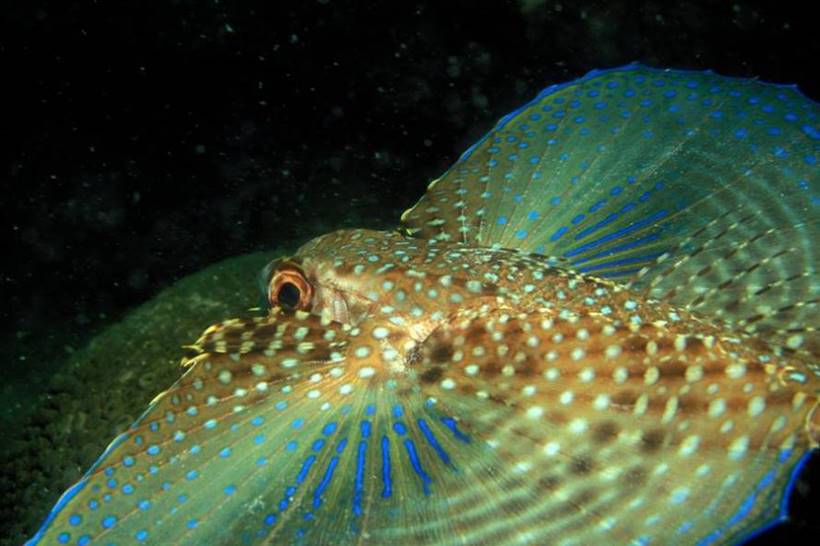In the deep, pitch-black waters, a mesmerizing creature, likely an octopus or cuttlefish, floats ethereally. The close-up photograph showcases its colorful, multi-hued body radiating shades of blue, green, yellow, and gray, with vibrant neon blue outlines giving it a glowing appearance. Its surface is further adorned with white spots and dots. At the center, a distinct black eyeball with a greenish-yellow iris stands out, adding to the mysterious allure of this aquatic being. The creature is surrounded by bubbles and particles, enhancing the underwater vibe, and though it's challenging to discern any distinct background elements, the possibility of coral or underwater flora subtly emerges. The overall effect is one of beautiful, vibrant colors reflecting ambient light, making the enigmatic sea creature shine brilliantly against the dark abyss.